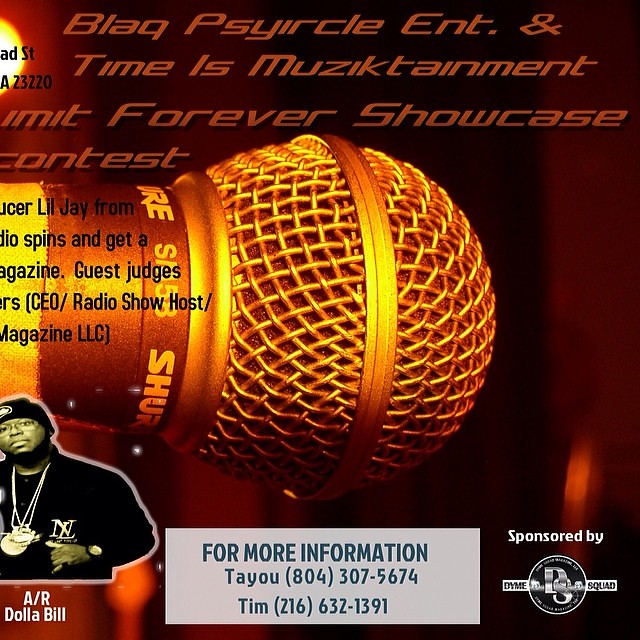The promotional poster for the "Blaq Psyircle Entertainment: Time is Musictainment - Umit Forever Showcase Contest" features an intensely zoomed-in image of the head of a microphone, illuminated with an orange-brown filter. The background is a blurred maroon wall. Central to the poster is the event title in brown and goldish text, though some details are obscured. Key visible text includes "Ad Street A23220" as part of the address, and mentions of "Lil' J from Spins" and a "magazine," alongside references to guest judges whose names are cut off. In the lower left corner, there's a photo of an African American man wearing metallic medallions, a black shirt, and a black knit cap, tagged with the subcaption "ARDOLLABILL". For more information, the contact details provided are Tayo at 804-307-5674 and Tim at 216-632-1391. The event is sponsored by "Dime Squad," whose logo is positioned at the bottom right corner of the poster.